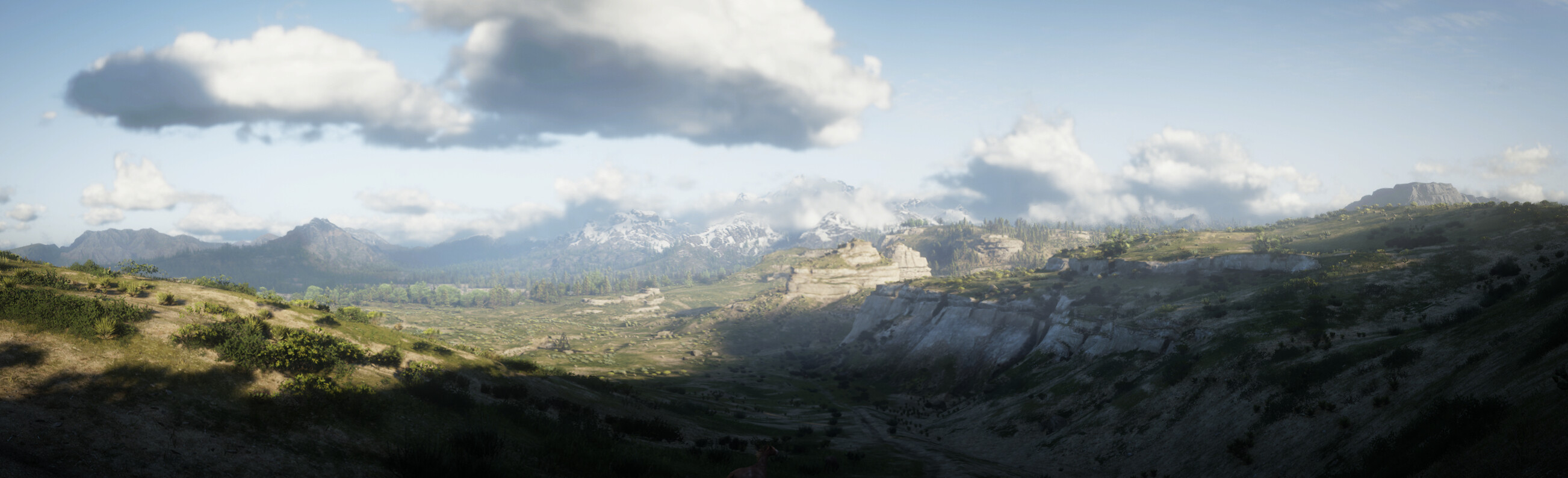This is a captivating and serene image of a vast and rugged mountain landscape, seemingly taken from a high vantage point, perhaps from someone who has climbed the terrain. The scene features a long, thin portrait showcasing the majestic great outdoors. To the left, there is a hill primarily composed of dirt with patches of vibrant green shrubbery. On the right, the landscape shifts to craggy rock formations. The middle of the image reveals a valley surrounded by mountains. In this valley, clusters of trees and a potential lake can be seen, indicated by a clearing without trees. The mountains continue into the background, with varying elevations, some adorned with pine trees and others capped with snow. Darker mountains loom in the distance to the left. The sky above is adorned with several high, fluffy clouds, including two particularly large ones in the upper left corner, their undersides tinged with grey shadows. The bright and clear day bathes the scene in sunlight, enhancing the natural beauty of the green terrain and rugged rocks. The horizon shows peaks that rise above some clouds, accentuating the vastness of the mountain range. The overall atmosphere of the photograph is one of peaceful isolation, untouched by human presence, encapsulating the essence of nature's grandeur.